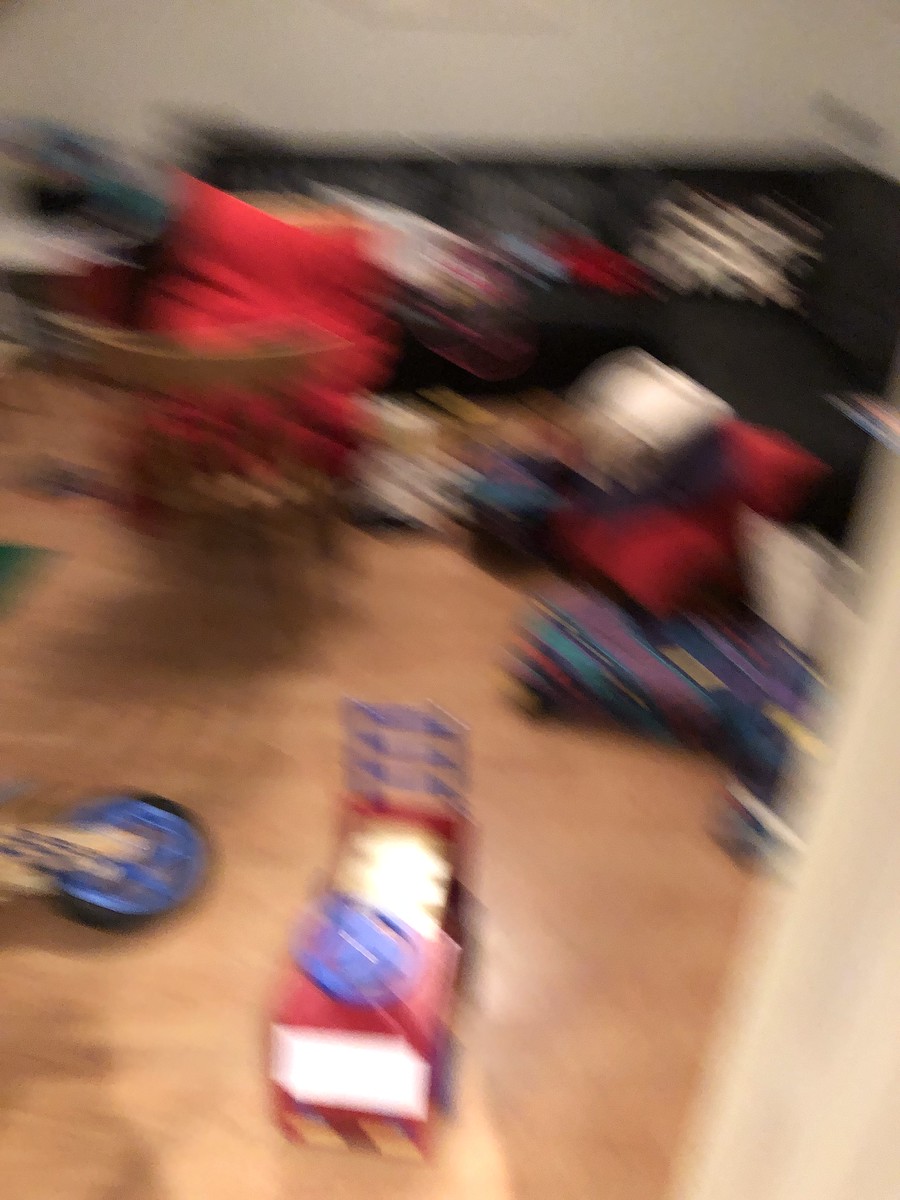This extremely blurry photograph in portrait format depicts the interior of a vibrant living room or a child's play area. Dominated by a wooden floor, the image shows a scene filled with colorful, child-friendly elements. At the center and in the foreground, a mix of furniture and toys are barely discernible due to the motion blur of the photograph. Notable details include a black couch cluttered with multiple cushions in colors like red, yellow, white, and blue. The floor is scattered with additional cushions and toys, including a toy fire truck. In the background, a black bookcase with striking diagonal white, red, and blue stripes stands out against a white painted wall. The blur and streaks across the image suggest it was taken hastily, capturing multiple colorful objects along the left and right sides of the room, including hues of green, pink, and purple among others. The overlapping details, streaks, and vivid colors hint at a lively, dynamic space dedicated to a young child’s activities.